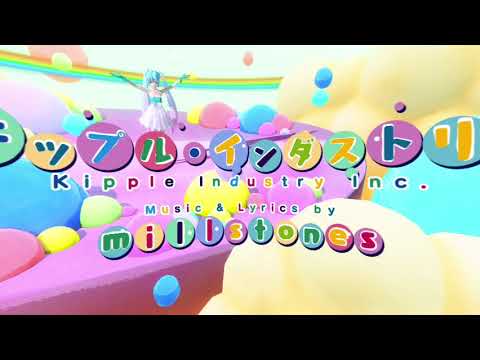This vibrant digital poster might be a splash screen for a video game, website, or video. The background is a colorful, festive scene featuring pastel-colored circles, ranging from pink, blue, and yellow to green, purple, red, and teal. The background also includes whimsical yellow clouds and a delicate rainbow set against a white sky.

At the center of the image stands a cartoonish anime girl with long, teal pigtails, dressed in a white outfit on a pink, candy-like platform. Her arms are open wide, giving an energetic and inviting gesture.

Text is prominently displayed across the image. At the very top center, the text "Kipal Industry Inc." appears in a playful array of colors, with each letter situated within a different bubble. Beneath that, the text "music and lyrics by" is written, followed by "M-I-L-L-S-T-O-N-E-S," with each individual letter placed inside its own bubble, resembling Japanese or other oriental symbols.

Framing the entire scene, there are thin, horizontal black and yellow strips at both the top and bottom of the image, adding a striking contrast to the vibrant and cheerful middle section.